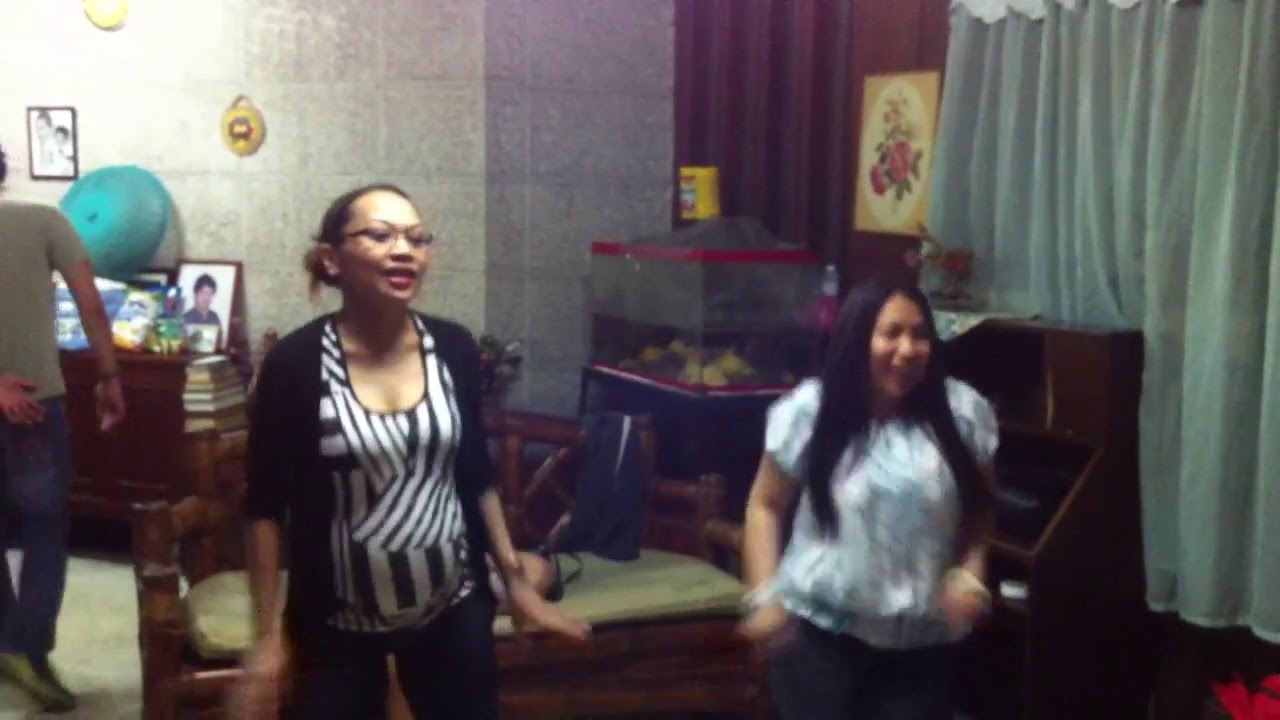In a modestly lit room with varied wall textures, ranging from large cinder blocks and white stucco to curtains in different colors (red, green, brown) and assorted paintings and photographs, two women stand prominently near a wooden bench. The left figure, taller and more mature, has her hair pulled back and wears glasses, along with a black and white top and black pants. She has her hands hanging down at her sides. The woman on the right, possibly a younger individual or child, is noticeably shorter, with long black hair cascading over her fluffy, frilly blue shirt. Both women appear to be in motion, possibly dancing or singing, evidenced by the blurred depiction of their hands, creating a sense of dynamic movement in the photo. In the background, partially obscured by the image's framing, a man in a green short sleeve shirt and jeans stands to the left, potentially playing a piano. The room’s eclectic decor, including wooden elements and hints of a church-like setting, suggests this might be a casual rehearsal space, perhaps for a church choir.